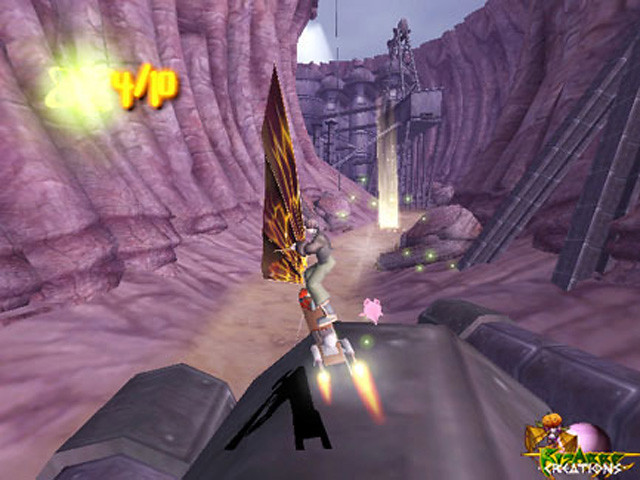The image is a screenshot from a video game that features a human figure riding a jet-powered sailboard through a narrow canyon with steep walls. The sail has a distinct triangular shape and is colored yellow and black. This figure is positioned above a large gray craft, moving over it with visible flames coming from the small jet engines on both sides of the board. In the distance, at the end of the canyon, a tall tower can be seen, contributing to the game's immersive environment. On the right side of the image, leaning against the canyon wall, are black linear items. Additionally, there is a logo and some text in the lower right corner, with the legible words "Creations" in white and a word in green that might be "KIZARE." The upper left corner displays the text "4/10" in yellow, which could indicate a scoring system or rating.